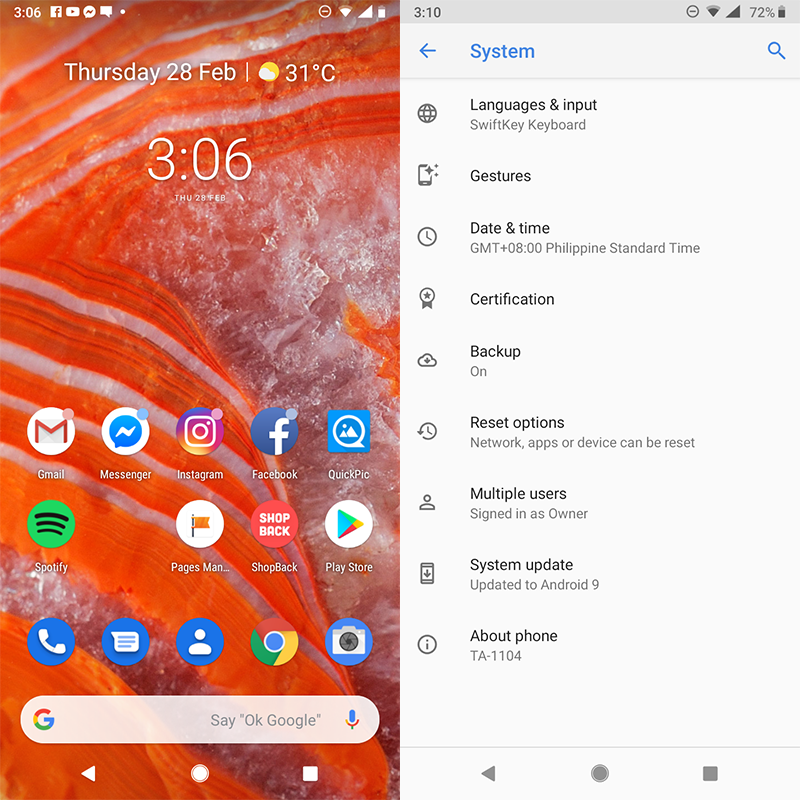A futuristic smart screen, dated Thursday, 24th of February, 2306, displays an array of icons including Gmail, Facebook Messenger, Instagram, Facebook, QuickPix, Spotify, Pages, ShopBack, and the PlayStore. Additional icons present are for calling, a comic book reader, Google Chrome, the camera, Google, a microphone, a sideways triangle, a dot, and a square. The screen also shows system options such as languages and inputs, keyboard gestures, date and time settings, a TNT Philippine Center Tank Certificate, backup and reset options, multiple user configurations, sign-in details, and system updates. At the bottom are essential navigation controls: a microphone, a sideways triangle, a circle, and a square.